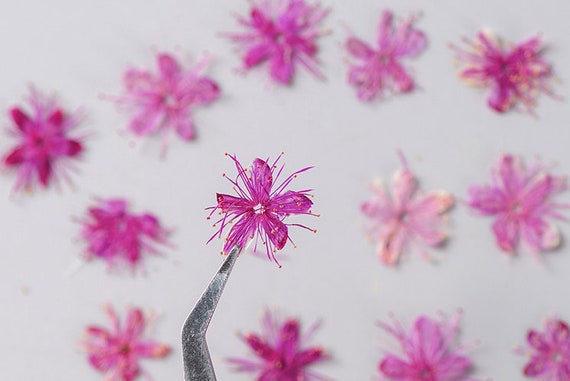The image captures an array of vividly colored flower petals, predominantly purple with a hint of pink, each arranged in star-like patterns. The primary focus is on a single set of five purple petals adorned with fine tendrils, which is being delicately held up for the camera by a pair of textured silver tweezers. This set is in sharp focus, allowing a clear view of the intricate details, including a small white cluster at its center. In the blurred background, additional sets of similarly styled pink, purple, and white petals are scattered across a white surface, contributing to a rich and textured floral scene.